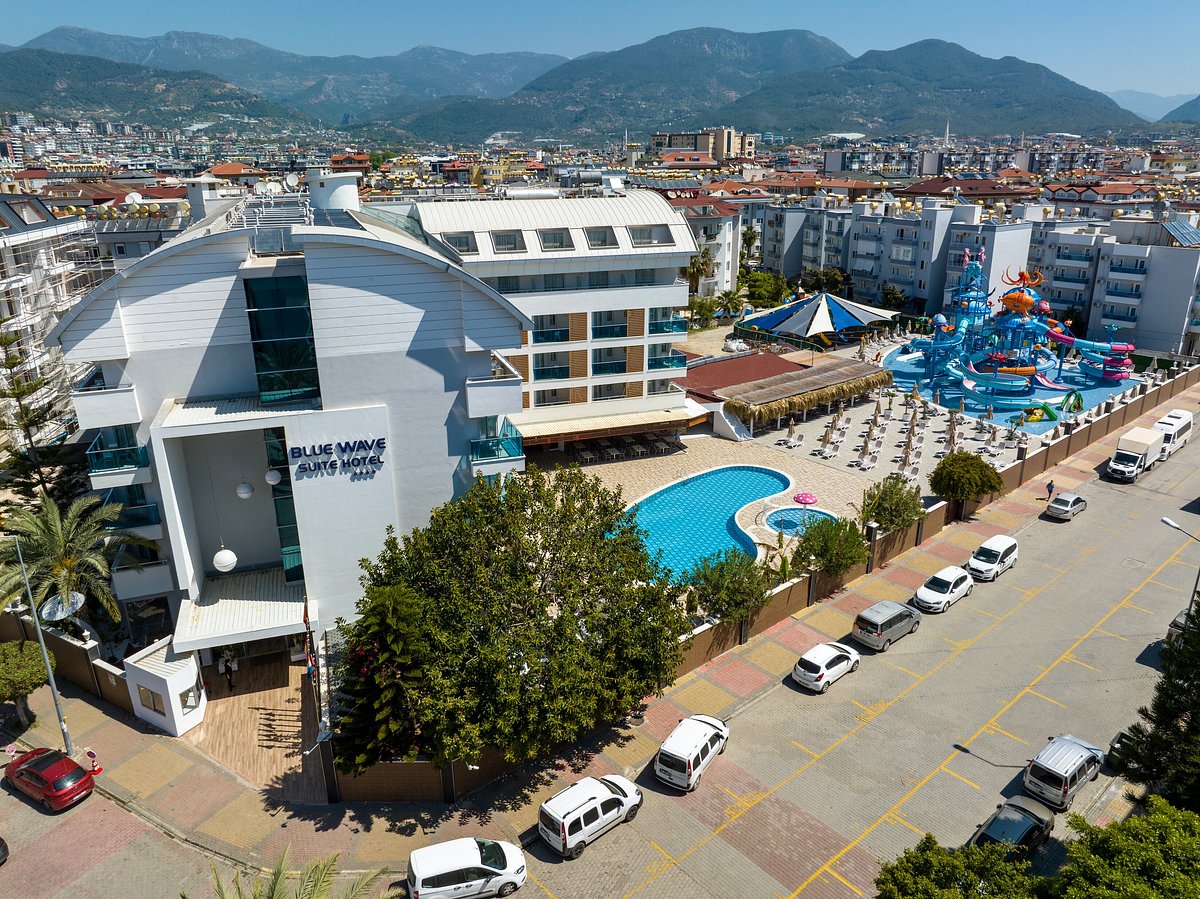The aerial view, likely captured by a drone, showcases a bustling cityscape nestled in a valley with distant mountains accentuating the horizon. Dominating the foreground is the modern Blue Wave Suite Hotel, recognizable by its distinctive glass facade and curved, half-cylinder roof. Encircling the hotel is a brick-walled recreational area featuring a well-laid-out pool complex, including a main pool, a water spray area leading into a smaller adjacent pool, and a large play area with various slides, evoking an aquatic fun center atmosphere. Numerous chaise lounges are strategically positioned beside what appears to be a bar with a palm tree motif. The scene is vibrant and crowded, with a line of white taxi vans and other vehicles parked right in front of the hotel, adding to the urban hustle. A big tree and a palm tree in the immediate vicinity further embellish the hotel's front area, while the backdrop reveals a dense sprawl of apartment blocks and stores under a slightly smoggy sky, highlighting the expansive nature of the city.